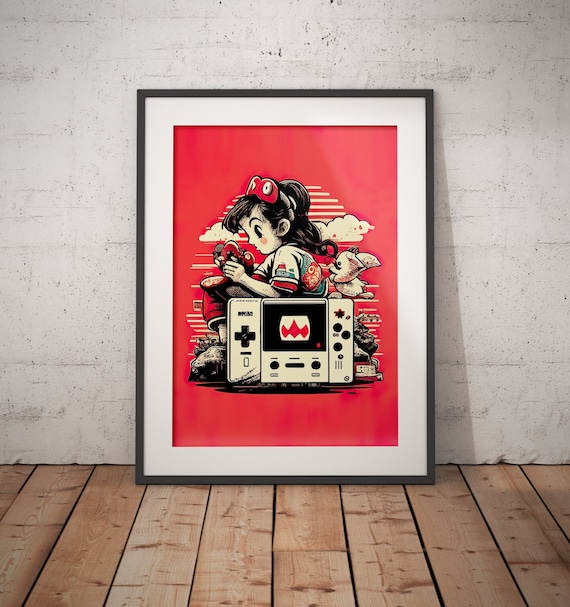A vertical, full-color photograph shows a framed print leaning against a wall on a wooden floor. The image features a simple, nearly black frame with a white matting. The floor, occupying the bottom 25% of the photo, consists of wooden boards with visible knots and vertical separations. Behind the frame, the concrete wall, painted a stuccoed gray, provides a minimalistic backdrop.

The framed print itself has a red background and portrays a young child in profile, their gender ambiguous. The child has dark hair cascading halfway down their back and wears goggles or a visor pushed up on their forehead. The child is engrossed in playing a handheld video game device, possibly a controller or a CB radio, while seated cross-legged. The illustration is predominantly in red tones, creating a striking visual against the minimalist setting.